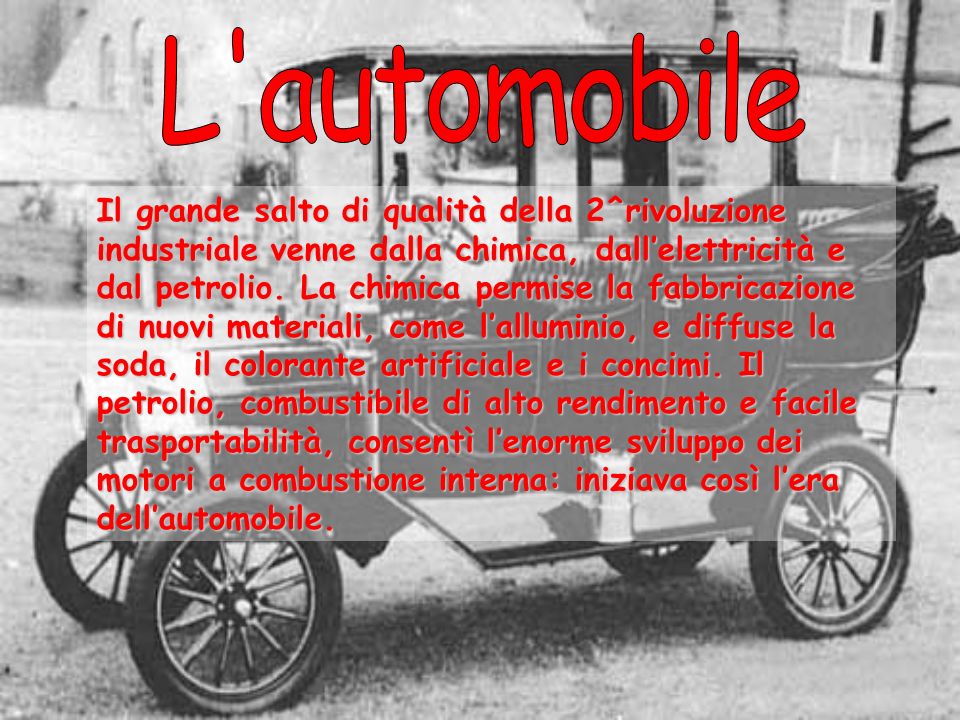The black-and-white photograph depicts an early automobile from the late 1800s or early 1900s, positioned centrally and facing left. The car has a thin structure with small wheels and a carriage-like back, resembling a modern golf cart. Overlaid atop the image is red text in Italian, with the title "L'automobile" at the top and an 8-9 line paragraph describing the importance and efficiency of the automobile. The text emphasizes industrial advancements through chemicals, electricity, and oil, highlighting the creation of new materials like aluminum and the production of consumables such as artificial colorants and soda. This image appears designed for educational or promotional contexts, showcasing the innovative quality and fuel-efficiency of early automotive technology.